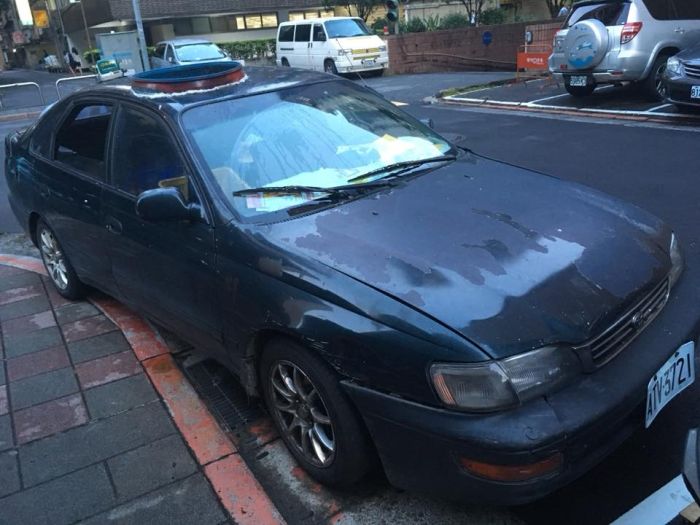The image depicts a worn-down, older model black or dark blue Japanese car, possibly a Honda or Toyota, parked awkwardly with its rear right tire on a red curbside. The car's paint is significantly faded and chipped, particularly on the hood, bumper, and sides, leaving shiny and smooth patches. Visible modifications include a red-ringed blue patch on the roof, likely covering a hole. The front bumper appears broken and partially fallen. The windshield reflects shine, and the wipers are running, suggesting recent rain. This scene unfolds on a wet asphalt road in a sleepy downtown or suburban shopping area, with wet patches visible on the dark-brick patterned sidewalk. Background elements include multiple parked vehicles—a silver SUV, a white van—and a gray building adorned with numerous windows and railings.